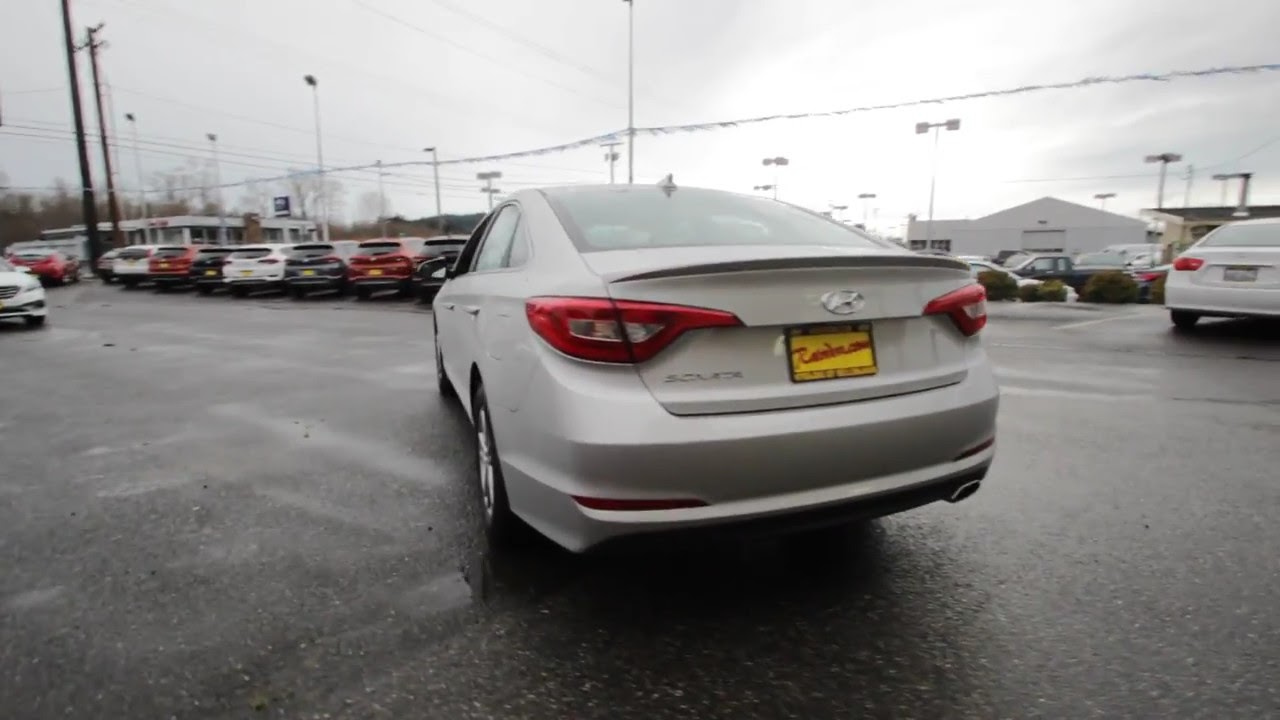The image captures an outdoor car lot, likely associated with a car dealership, set against an overcast sky. The focus is on a central silver Hyundai vehicle, identifiable by its logo, which is either backing up or turning, with its red taillights glowing. This car lacks a visible registration plate but has a dealership plate with ".com" partially visible. Surrounding the Hyundai are several other vehicles lined up, including white, black, red, and blue SUVs, suggesting that this is a used car lot. The background features multiple buildings, including an office or showroom to the right and another structure with a car manufacturer's logo on the far left. Trees with no leaves and numerous power lines and loudspeakers frame the scene, contributing to the autumn or early winter setting. The entire area is paved with asphalt, and the lot is organized with parking spaces marked out on both sides.